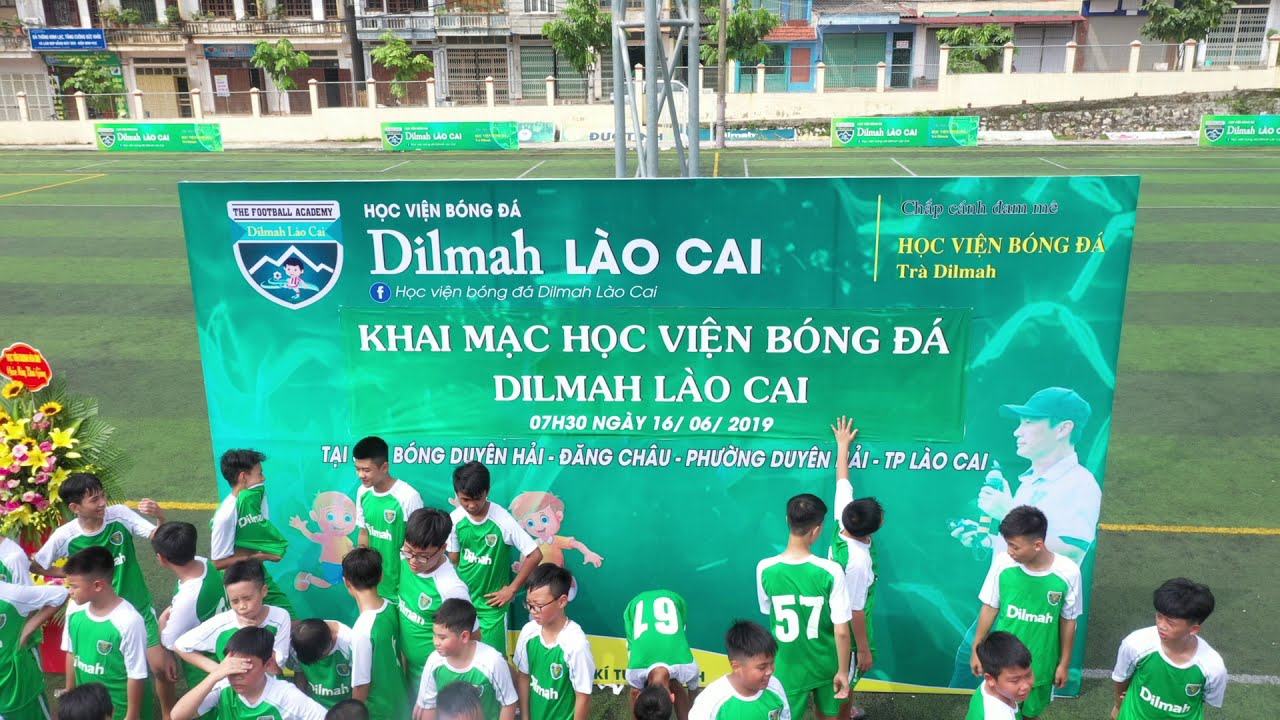A vibrant and lively scene captures a children's soccer team, seemingly aged around 11 or 12, clad in green and white jerseys emblazoned with the name DILMAH (D-I-L-M-A-H) on the front and numbers on the back. These young players, likely part of an Asian youth soccer tournament, interact animatedly amongst themselves. The setting is an outdoor soccer field, bordered by multiple event banners inscribed with Vietnamese text, hinting at the tournament's location. Dominating the background is a large vinyl banner featuring the title "Dilmahalaukai Khaymakhokvienbongda Dilmahalaukai" and a logo in the top left corner. Large bouquets of yellow and pink flowers to the left add a festive touch to the environment. In the farther background, a grassy field extends towards some building structures, reinforcing the bustling and competitive atmosphere of the event. A visible date on one of the signs, June 16, 2019, adds a temporal context to this energetic snapshot of youth sportsmanship and cultural celebration.